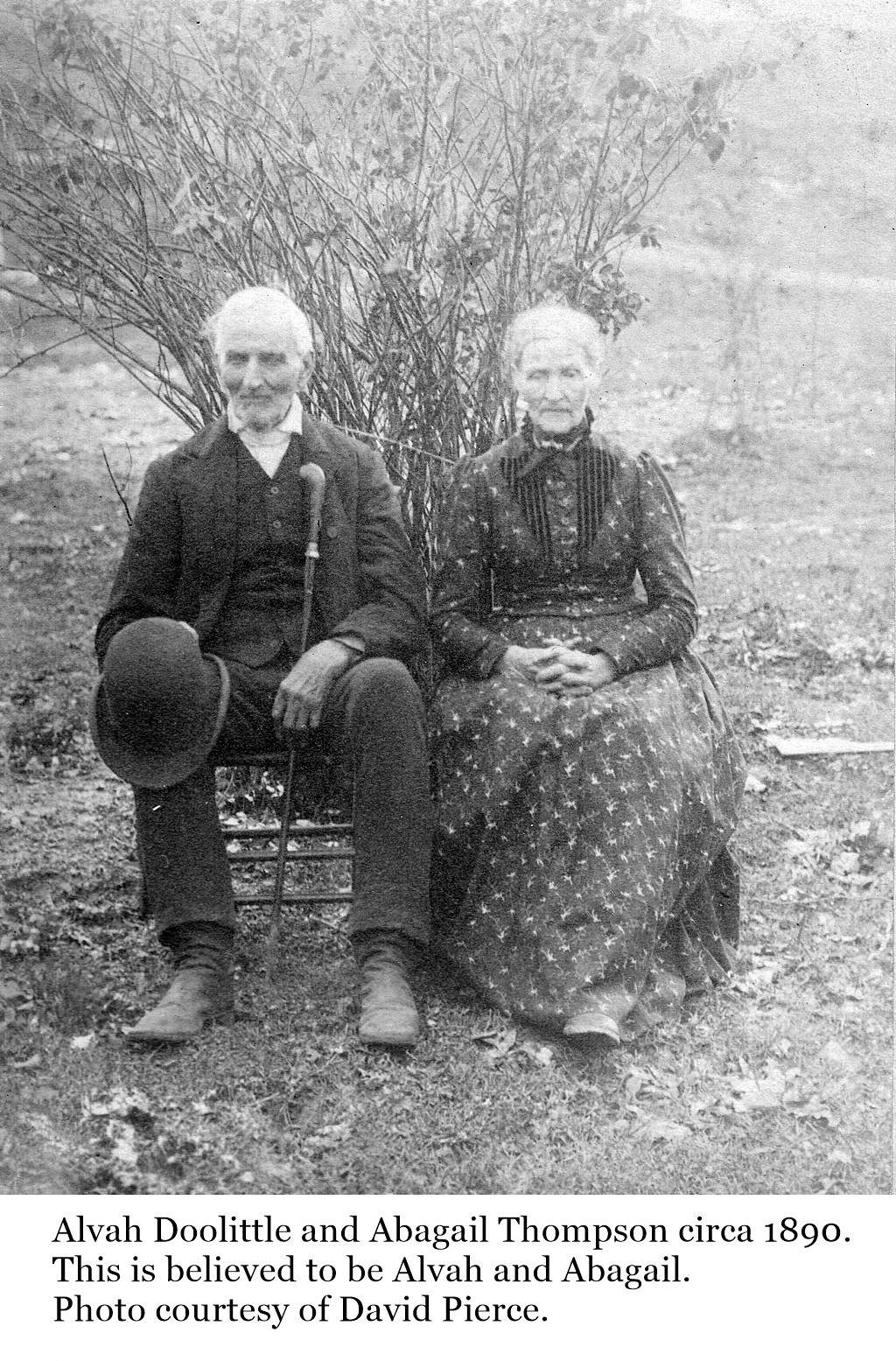In this black and white photograph, an elderly couple, Alva Doolittle and Abigail Thompson, sit together in a grassy outdoor setting, with leaves scattered around and trees visible in the background. The middle of the day light illuminates the scene, highlighting the period clothing of both individuals—Alva in a suit and pants, and Abigail in a dress—as they pose directly at the camera. The image, likely taken around 1890, is credited to David Pierce. Text at the bottom of the photograph confirms the identity and date, and the overall quality suggests the age of both the photo and the subjects.